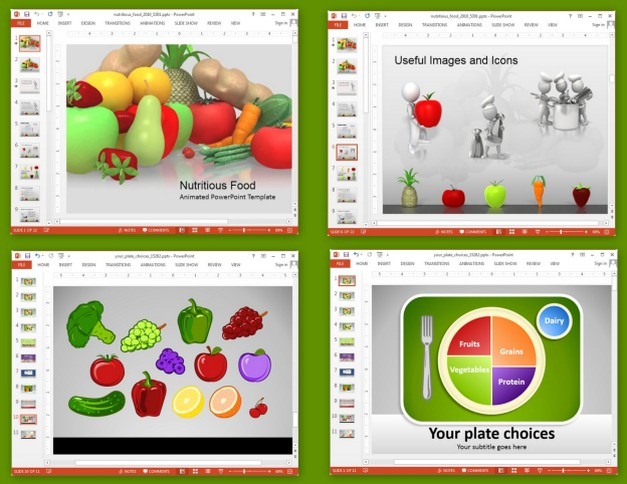The display is a set of four computer-generated images showcasing a nutritious diet and meal planning, formatted as PowerPoint slides. 

In the upper left, the first slide is labeled "Nutritious Food Animated PowerPoint Template" and features a variety of vibrant fruits and vegetables, including strawberries, a pear, an apple, a pineapple, carrots, tomatoes, asparagus, and beans. The background is grey, and smaller, indecipherable template designs line the left side.

The upper right slide titled "Useful Images and Icons" displays simple stick figure characters interacting with fruits and vegetables. One character holds a red apple, while another trio stirs a pot. Fruits such as an apple, a pineapple, a pear, a strawberry, and a carrot are shown on a table.

In the bottom left, the third slide, also set against a grey background, showcases animated illustrations of assorted fruits and vegetables like broccoli, grapes, tomatoes, green and red peppers, lemons, and oranges, though it lacks a clear label due to small text.

The bottom right slide, marked "Your Plate Choices. Your subtitle goes here," depicts a divided plate for balanced meal planning. It allocates sections for fruits, vegetables, grains, and protein, accompanied by a fork on the left and a dairy cup to the upper right, encouraging well-rounded nutrition.